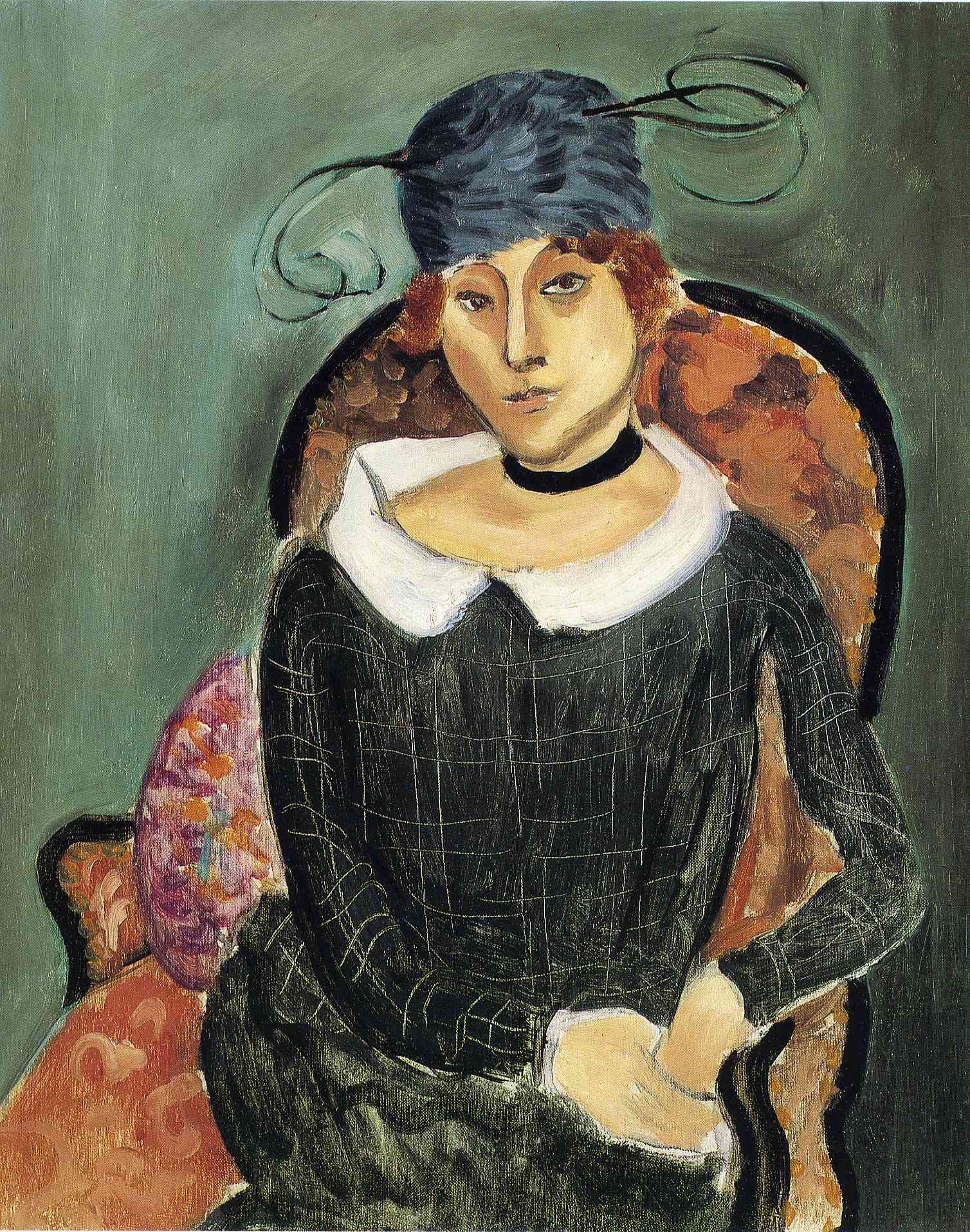In this distinctive, yet somewhat peculiar painting, a middle-aged woman is seated in a visually captivating chair, bathed in a unique blend of realism and artistic exaggeration. Her red hair, neatly tucked under a gray hat adorned with feathers and large ribbons, adds a flamboyant touch to her appearance. She wears a black choker necklace tightly around her neck, paired with a white-collared, long black dress that intriguingly includes a plaid pattern with white outlines. The setting features an olive green background that contrasts with the vibrant colors of the chair she occupies. The chair itself is a plush, large piece, primarily orange with a black frame, accentuated by a multicolored cushion or pillow in shades of purple, orange, green, and red. The painting, which is vertically oriented, captures the woman from her thighs to the top of her head. Seated with her hands resting together on her lap, she exudes a soft, welcoming smile and a gentle stare, adding to the painting's allure. The overall palette includes hues of pink, purple, orange, black, white, gray, olive green, blue, and red, offering a rich visual experience.